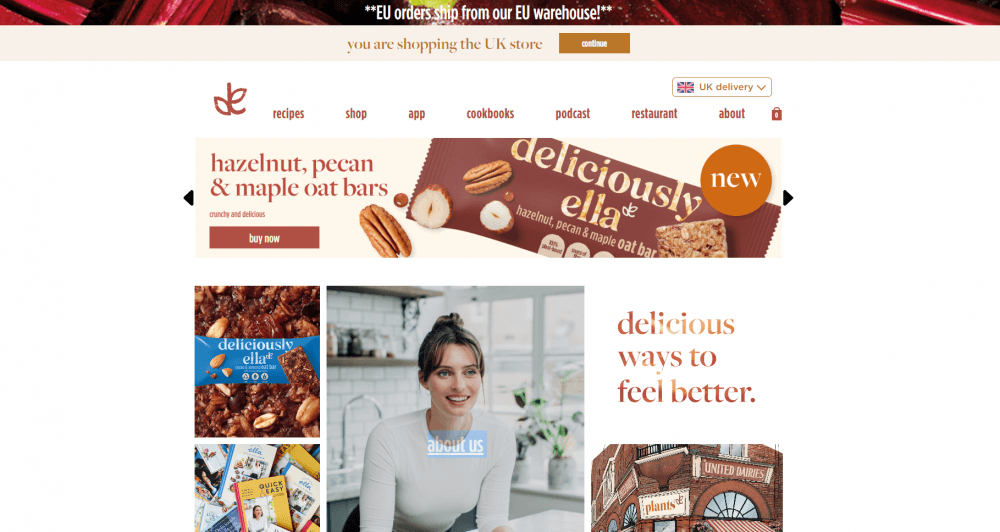The image displays a section of a website with a vibrant and structured layout. 

At the top, a banner announces "EU order shipped from our EU warehouse" set against a distinctive background featuring diagonally oriented stripes in red, white, and pink. Immediately below, a message reads "You are shopping at the UK store," accompanied by a brown rectangular button. 

The navigation bar contains a red logo depicting two leaves on the left, followed by links labeled "Recipes, Shop, App, Cookbooks, Podcast, Restaurant, About," and an icon resembling a shopping bag, all rendered in dark red.

Below the navigation bar, a featured product is highlighted: "Hazelnut, Pecan, and Maple Oat Bars." A "Buy Now" prompt is next to an image of the product packaging, which displays the brand name "Deliciously Ella" in gold text, alongside a dark orange circle labeled "New."

Further down, four smaller images are presented. The top left image shows a product named "Deliciously Ella" in blue packaging, surrounded by various nuts. Beneath this, an image depicts multiple yellow and white book covers. To the right of these, an image features a smiling woman wearing a light gray shirt, positioned in what appears to be a light gray kitchen. The final image on the far right displays text with a mixed dark red and light brown color scheme, proclaiming "Delicious ways to feel better," and at the bottom, an illustration of a building with the word "Plants." The entire layout is set against a clean white background.